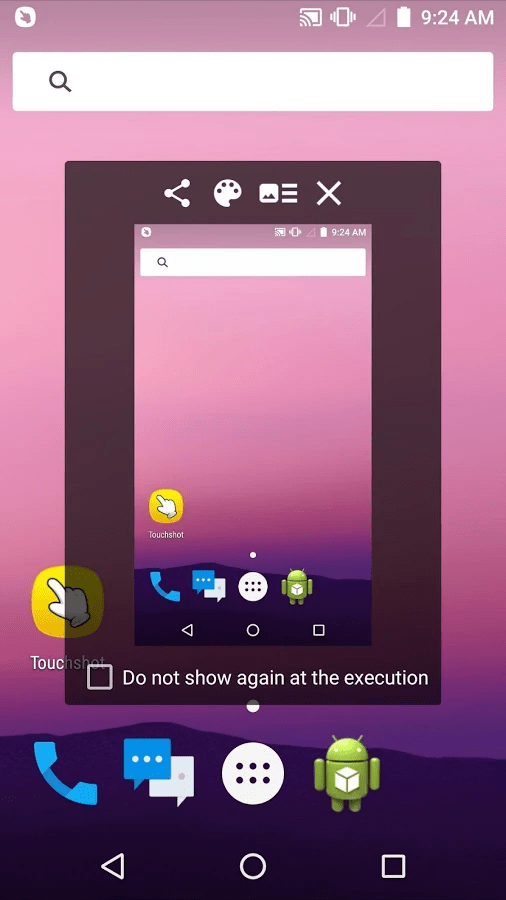The mobile home screen on an Android phone is meticulously detailed. At the very top, there is a long, narrow rectangular search bar adorned with a magnifying glass icon. The status bar displays several icons, including an active cast symbol, a vibrate notification indicating that the phone is set to vibrate, a faint network signal icon, a fully charged battery icon in white, and the current time, which is 9:24 a.m., positioned in the right-hand corner.

At the bottom of the screen are the three navigational buttons characteristic of Android devices: the back button, the home button, and the multiple or previous apps button. The home screen appears as a miniaturized screenshot, showing several app icons and a message overlay.

The visible app icons include the Touch Shot app, the Phone app, the Text Messages app, the All Apps button, and an Android app represented by an Android figurine icon. Additionally, overlaying the screenshot is a phrase that states "Do not show again at the execution" with a check box next to it, which can be selected to prevent this message from appearing in the future.